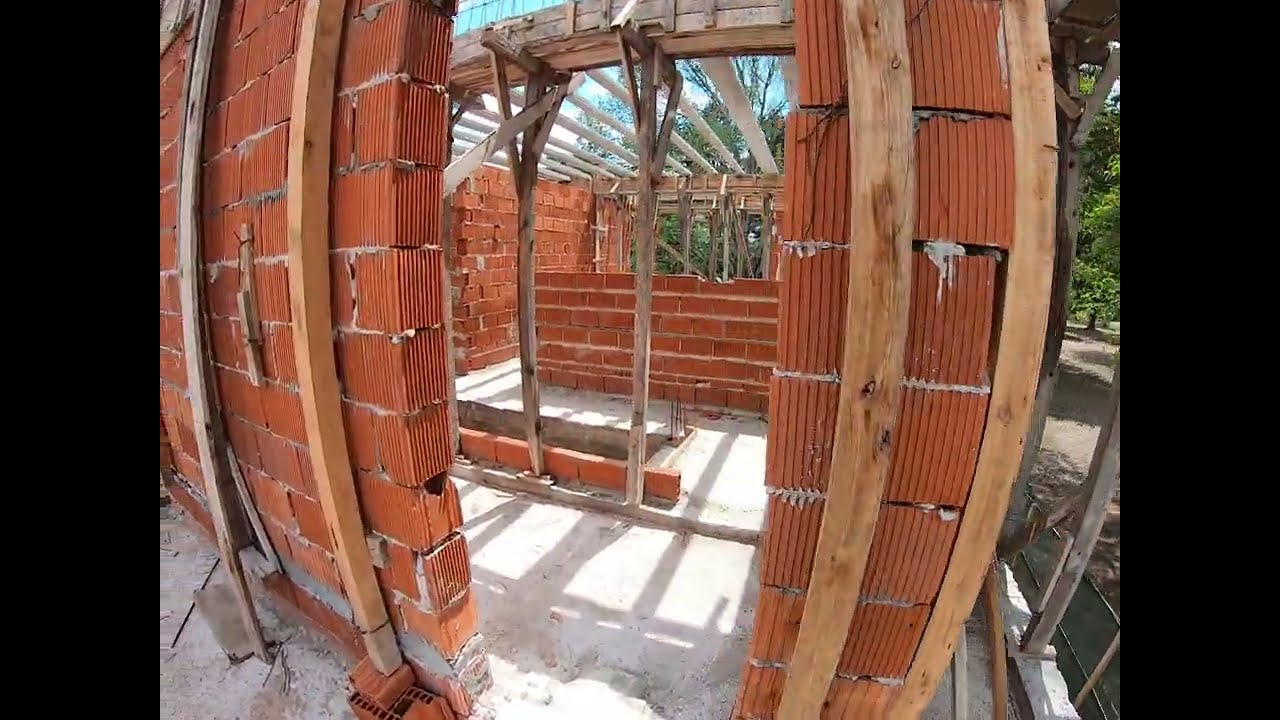This horizontally aligned rectangular image captures the exterior view of an unfinished construction project. The picture features a thick black border on the left and right sides, creating a frame for the scene. The structure in the image, which appears to be a house, is built from a combination of wood and distinctive red-brown bricks with white grout. The central focus of the picture is a half-completed brick wall. Above it, wooden boards laid across the top form the initial framework for the ceiling, with gaps revealing a blue sky dotted with white clouds.

The scene is set on a plain concrete ground, suggesting an early stage of construction, possibly just the foundation or slab floor. The building materials are visibly varied in finish; some areas of the grout are clean and precise, while others appear more haphazard, with excess running down between the bricks. The construction site looks active yet incomplete, with wood pallets or pillars supporting the precariously placed ceiling boards. In the background, the boundaries of the construction site blend into a natural setting with trees offering a touch of greenery. The overall look is slightly curved or distorted, giving a subtle fishbowl effect to the image.